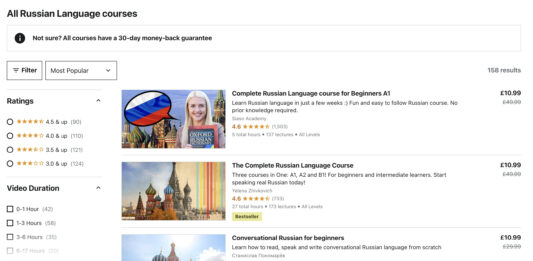The image is primarily a white screen featuring a structured layout for navigating Russian language courses. In the top-left corner, there is black text reading "All Russian Language Courses." Below this, there is a small outlined box containing a black circle with a white "i" information icon and the message, "Not sure? All courses have a 30-day money-back guarantee." 

Below this section, there are two interactive boxes: one labeled "Filter" and the other labeled "Most Popular" with a downward-pointing arrow. Further down on the left side of the screen, there are options for "Ratings," accompanied by a selection of star levels and another arrow. This is followed by a "Video Duration" section, which lists various time options.

Occupying the middle to right portion of the screen are images and video thumbnails depicting different areas of Russia. One of these images features a lady with a speech bubble. Each of these visuals is accompanied by descriptions and prices, which appear to be clickable for more information.